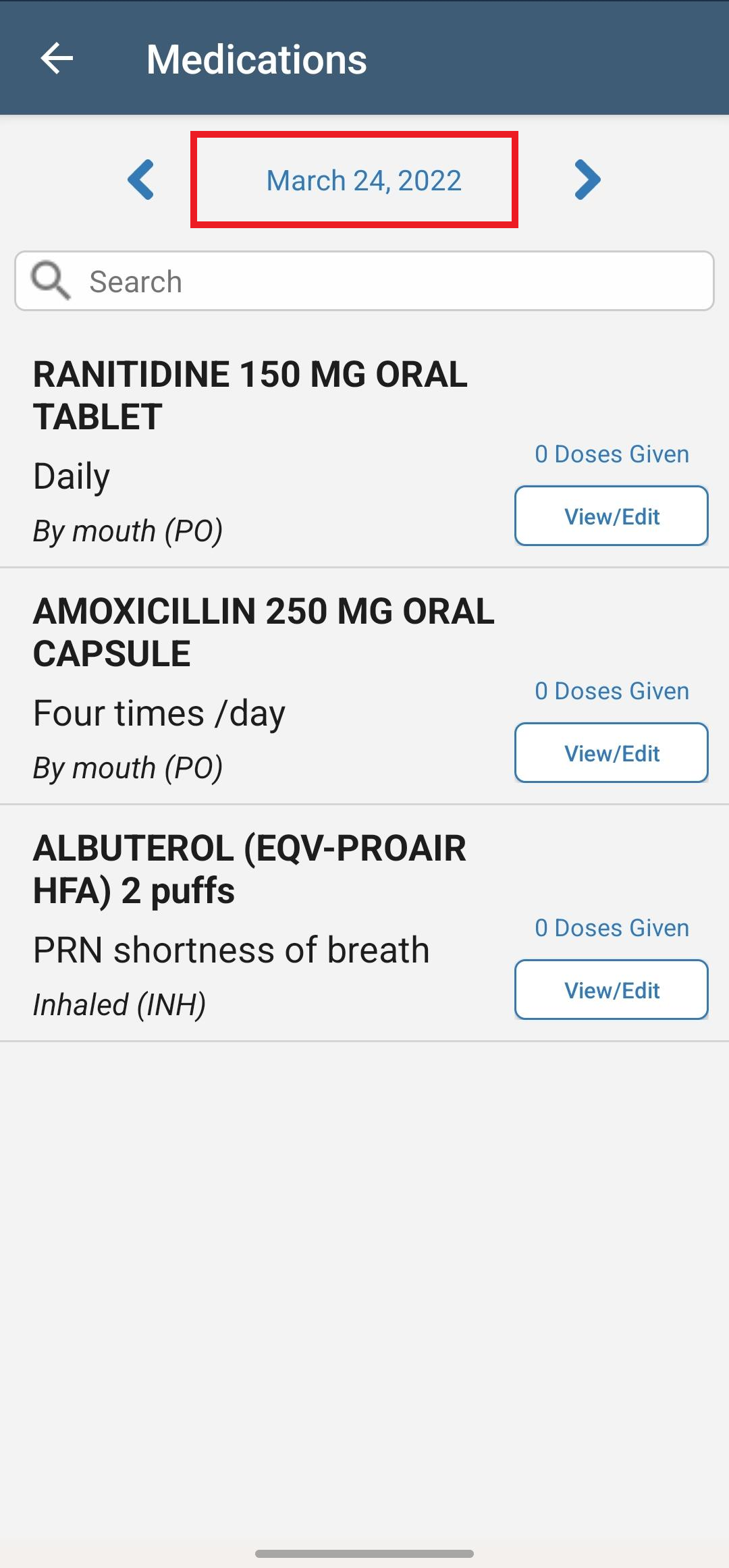This image is a detailed screenshot of a medication table, characterized by a structured, text-heavy layout on a gray background.

At the very top of the image, there is a blue box containing the title "Medications" in white text, accompanied by a left-pointing arrow.

Below this header, the gray background continues, displaying a blue arrow pointing to the left. Adjacent to the arrow is a red-outlined box with the date "March 24, 2022" written in blue text, followed by a right-pointing arrow.

Immediately below, a white search bar is present with the placeholder text "Search" in gray, accompanied by a gray magnifying glass icon.

The main content starts with the first medication entry:
- "RANITIDINE 150 MG ORAL TABLET" (all in uppercase) in black text.
- Below it, "daily" in lowercase black text.
- Further, "by mouth (PO)" appears in black within parentheses.
- To the right, "0 doses given" is displayed in blue text.
- A blue-outlined white text box containing "View/Edit" in blue is positioned next to the dosage information.
- This entry is separated from the next by a light gray line.

The second medication entry follows a similar format:
- "AMOXICILLIN 250 MG ORAL CAPSULE" (all uppercase) in black text.
- Below, "4 times/day" in lowercase black text.
- Further, "by mouth (PO)" within parentheses in black.
- To the right, "0 doses given" is mentioned in blue.
- A blue-outlined white text box with the words "View/Edit" in blue text appears next to this entry.

The third medication entry at the bottom of the list:
- "ALBUTEROL" (uppercase) followed by "(EQV-PROAIRHFA)" and "(2 puffs)" still in uppercase black text.
- Below, "PRN" remains in uppercase black text, followed by "shortness of breath" in lowercase.
- Further, "inhaled (INH)" within parentheses in black text.
- Similarly to previous entries, "0 doses given" is in blue.
- A blue-outlined white text box reading "View/Edit" appears to the right.

At the bottom center of the screenshot, a dark gray line is visible, adding a final element to the structured layout.